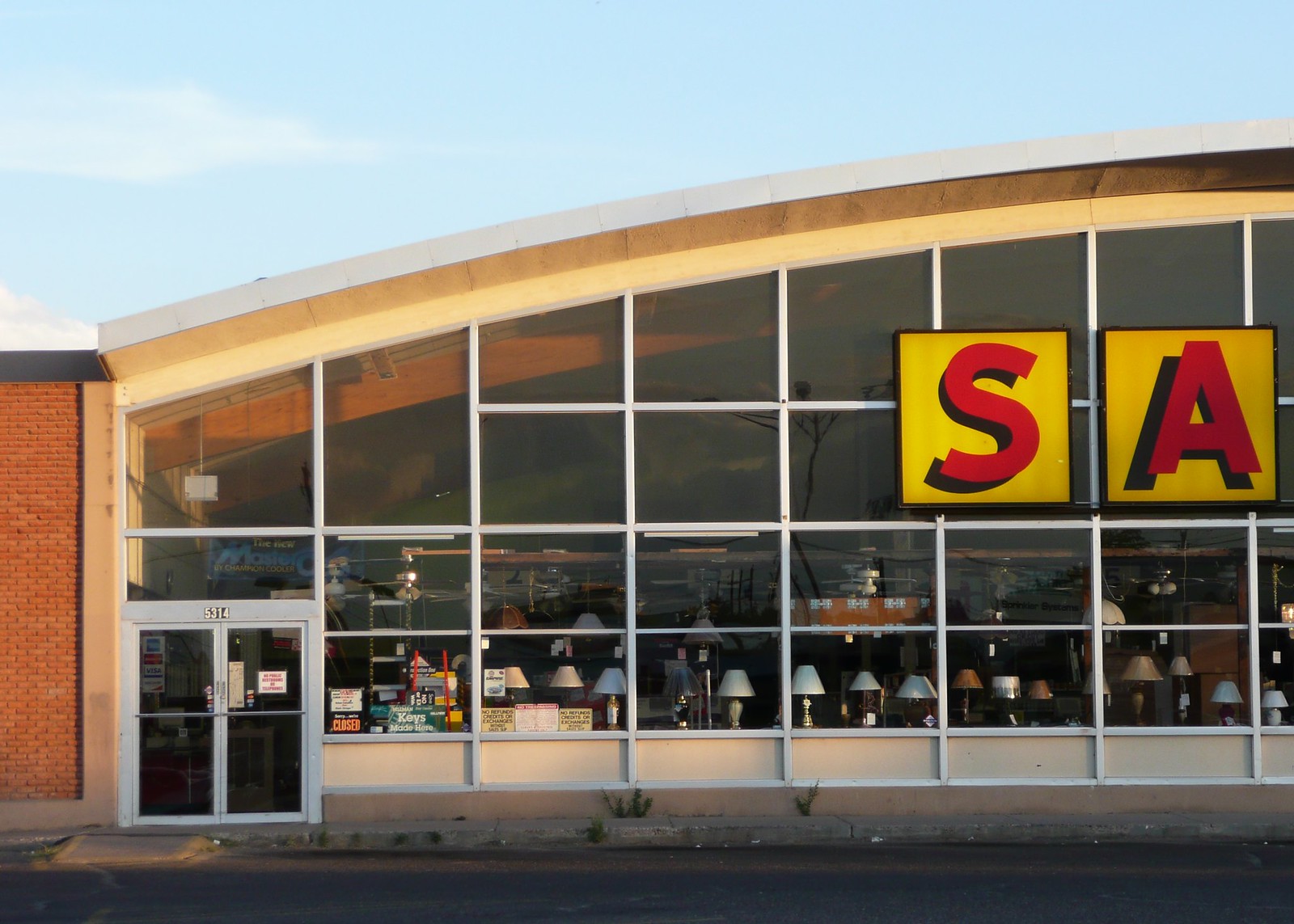A detailed photograph captures the façade of a brick hardware store with a prominent glass front. Through the expansive windows, an array of lamps is beautifully showcased, their various designs gleaming in the sunlight. Hanging ceiling fans are also visible towards the back of the store, adding to the store’s display of home fixtures. Above the windows, a yellow sign with the partially visible red letters "S" and "A" casts a shadowed outline against a yellow square. To the left of the glass frontage, two doors mark the entry point into the store. It is a bright, mostly sunny day, with a clear blue sky dotted with a few clouds. In the foreground, an empty parking lot stretches out before the store, providing an unobstructed view of the building's inviting entrance.